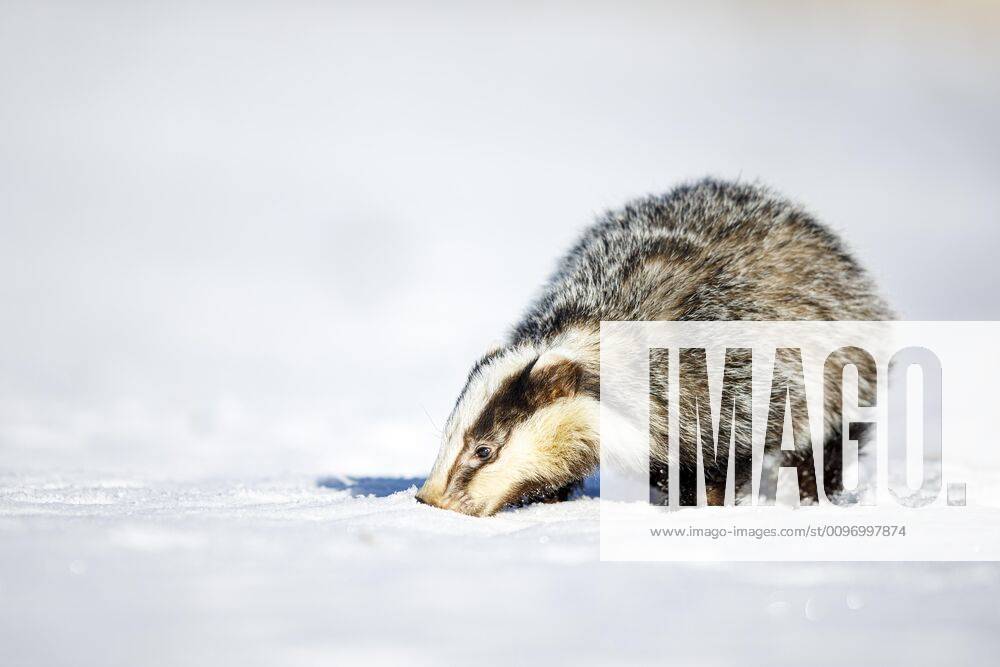In this photo set in a snowy landscape, the entire scene is enveloped in a cold, wintery atmosphere. The top half of the horizontal image displays a light gray, almost white sky. Just a bit past the halfway mark, the background bleeds into more distinct white streaks, eventually meeting the obviously snow-covered ground at the bottom. Positioned slightly right of center on this snow-covered ground is a furry animal with a distinctive appearance. Its head, facing to the left, is predominantly white, adorned with a black stripe running from its eye toward the back. The body of this small, likely weasel-like mammal, is roundish and features a mix of dark brown, black and white fur, blending seamlessly into the snowy surroundings as its nose touches the ground. Overlapping part of this picturesque scene, coming from the right side and positioned a little lower than the middle of the image, is a semi-transparent white rectangle watermark. The watermark partially obscures the animal's lower body from the head back. Within this rectangle, in transparent letters that allow the background to show through, are the characters "IMAGO". Beneath these letters, in smaller gray text, is the website "www.imagoimages.com" followed by a string of alphanumeric characters. The combination of the natural and the digital elements creates a unique and detailed visual narrative.